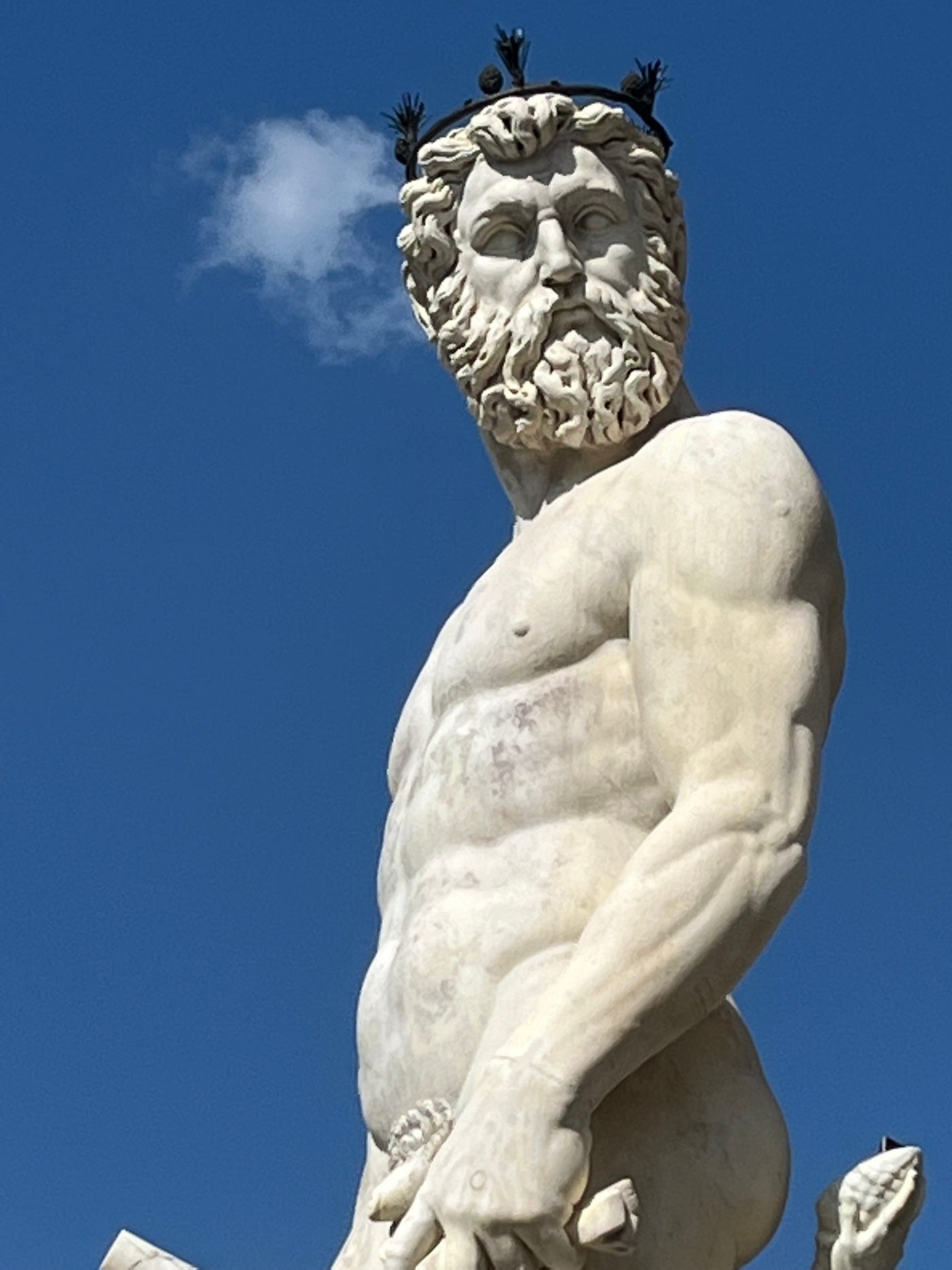In this striking portrait-oriented photograph taken from a low angle, we gaze upwards at a majestic white marble statue of what appears to be a Greek god. The statue is set against a radiant blue sky, with a single, wispy white cloud floating in the top left corner. The detailed shot captures the statue from the bottom of its buttocks upwards, with the muscular, naked form prominently displayed. The god's developed arms, chest, and abdomen showcase finely carved ridges, exhibiting impressive artistry.

The statue's body faces to the left, while the head, adorned with an intricate crown featuring small upward-pointing tassels, turns over the left shoulder to glance downward towards the camera. His face is framed by a luxurious mass of curly hair that merges seamlessly into a full, curly beard and mustache. In his left hand, lowered by his thigh, he holds an object that is partially obscured and cut off from the frame, adding an element of mystery. There's also an indistinct feature behind him, partially visible but not entirely clear. The photo's composition, with its rich blue sky and the carefully sculpted features of the statue, highlights the serene yet powerful presence of this classical figure.